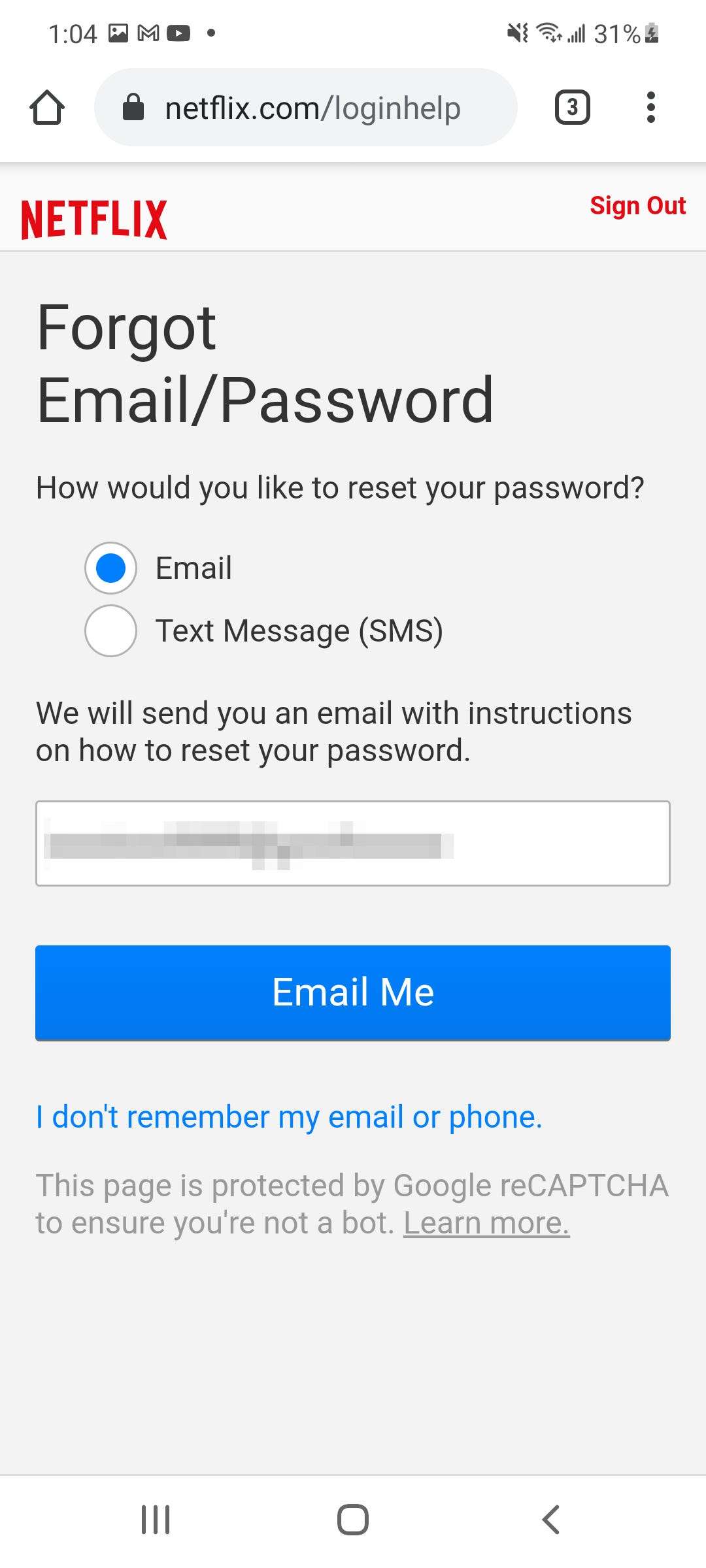The image is a screen capture from a mobile device displaying the Netflix login help page. At the top left corner, it shows the time "1:04." Surrounding the time are various system icons typically seen on a mobile interface. Directly below, the web address bar reads "netflix.com/loginhelp" in black text on a white background.

Centered on the page, bold red text spells out "Netflix." Adjacent to this, also in red, is a "Sign Out" option located on the top right. Beneath these headings, the background changes to an off-white hue. Prominently displayed in bold black text on this off-white strip is the phrase "Forgot Email/Password." Below this, in smaller black text, is a guiding question: "How would you like to reset your password?" 

Underneath this prompt, two radio button options are provided for resetting the password. The selected option is marked by a blue circle next to the word "Email."

This detailed depiction captures the layout and specific features of the Netflix login assistance page as seen on a mobile device.